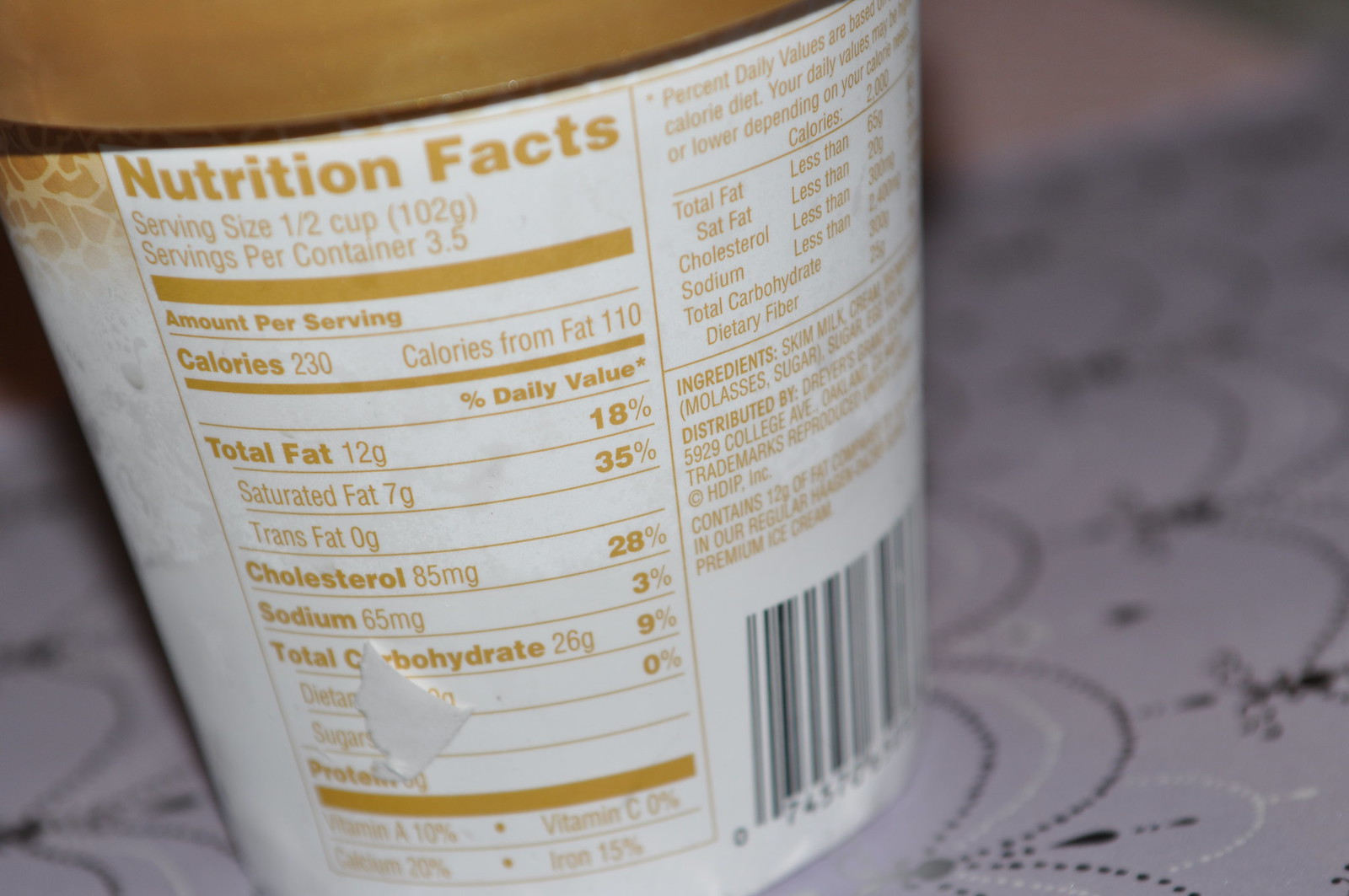This detailed close-up photograph captures the nutritional facts on the back of a small, white paper ice cream carton, reminiscent of a Ben & Jerry's container, with a goldish yellow lid. The focus is on the white label showcasing nutrition facts in yellow text, revealing a serving size of a half cup with 3.5 servings per container. The label details that each serving contains 230 calories, 12 grams of total fat, 65 milligrams of sodium, and 28 grams of carbohydrates, among other nutritional values. The surrounding area includes a white table with a decorative tablecloth featuring circular, bead-like designs. The carton also lists all the ingredients and has a UPC label. The absence of visible branding suggests that rotating the carton could reveal the brand name. The ice cream visual and detailed nutritional content form the central focus of this image.